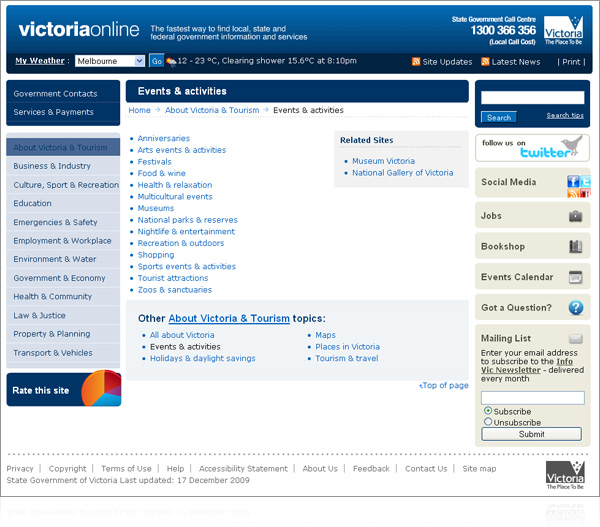The image features a white background with a prominent blue header at the top. Below the header, there is a blue box with white text stating "Victoria Online" and "The latest way to find local, state, and federal government information and services." The section also presents the State Government Call Center contact number.

In the center of the image, a white square with the word "Victoria" is displayed, followed by a dark blue box labeled "My Weather" with a search box where "Melbourne" is entered, adjacent to a blue "Go" button. Below this, news updates and the latest announcements are highlighted in orange boxes. There is also a print option indicated.

On the left side, a dark blue sidebar contains links to "Government Contacts," "Services," "Payments," and a comprehensive list of navigable items. A blue box beneath these links invites users to "Rate This Site" and features a pie graph in orange, blue, red, and purple.

Central to the layout is another blue box entitled "Events and Activities," which provides a detailed list of happenings. Further details about "Victoria" and "Tourism Topics" are enumerated with bullet points marked by asterisks.

On the right side, a blue box fills the area with a search box and prompts to "Follow Us on Twitter." Below, options for "Social Media," "Jobs," "Bookshop," "Events Calendar," and a "Got a Question" section are available. There is also a mailing list feature for users to subscribe or unsubscribe, presented with a submit button.

Finally, at the bottom of the image, privacy and copyright information is provided in a purple box featuring the word "Victoria."